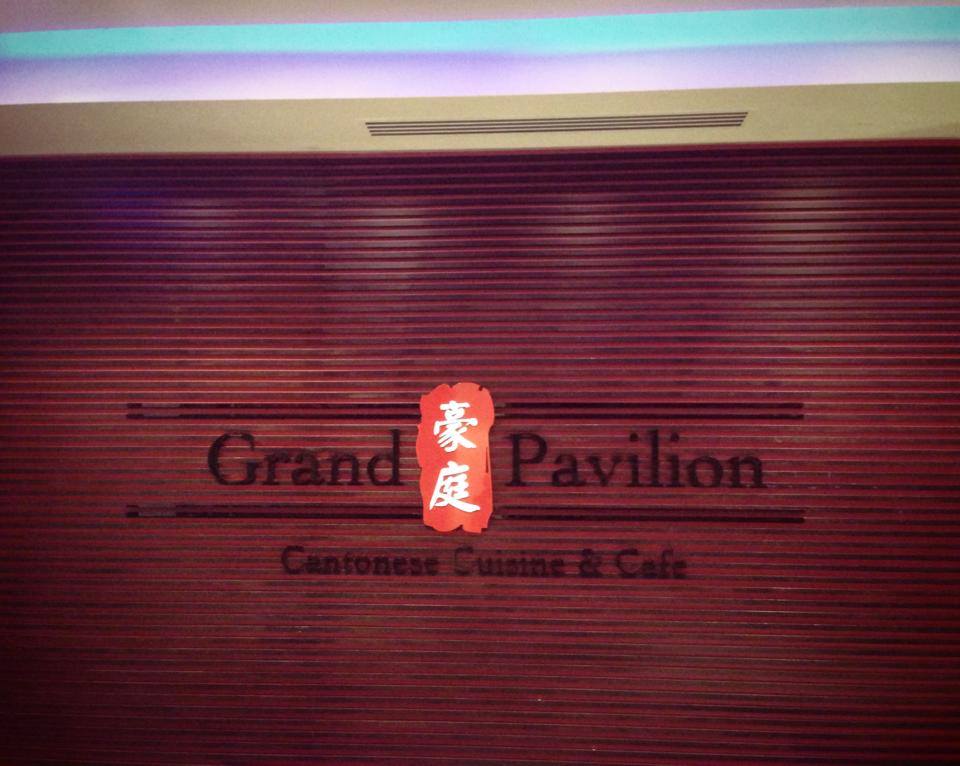The image depicts a detailed and vibrant logo on the side of a horizontally slatted wooden wall. Centered on the wall is the text "Grand Pavilion" in bold black letters, flanked by two horizontal black bars above and below. Between the words 'Grand' and 'Pavilion,' there is a prominent red emblem with two vertically stacked white Chinese characters. Below the main text, the words "Cantonese Cuisine and Cafe" are inscribed in black, offering a clear indication of the establishment's culinary focus. The wooden wall's distinct horizontal grain is complemented by a white ceiling above, which features an air conditioning vent and is subtly illuminated by blue lighting.